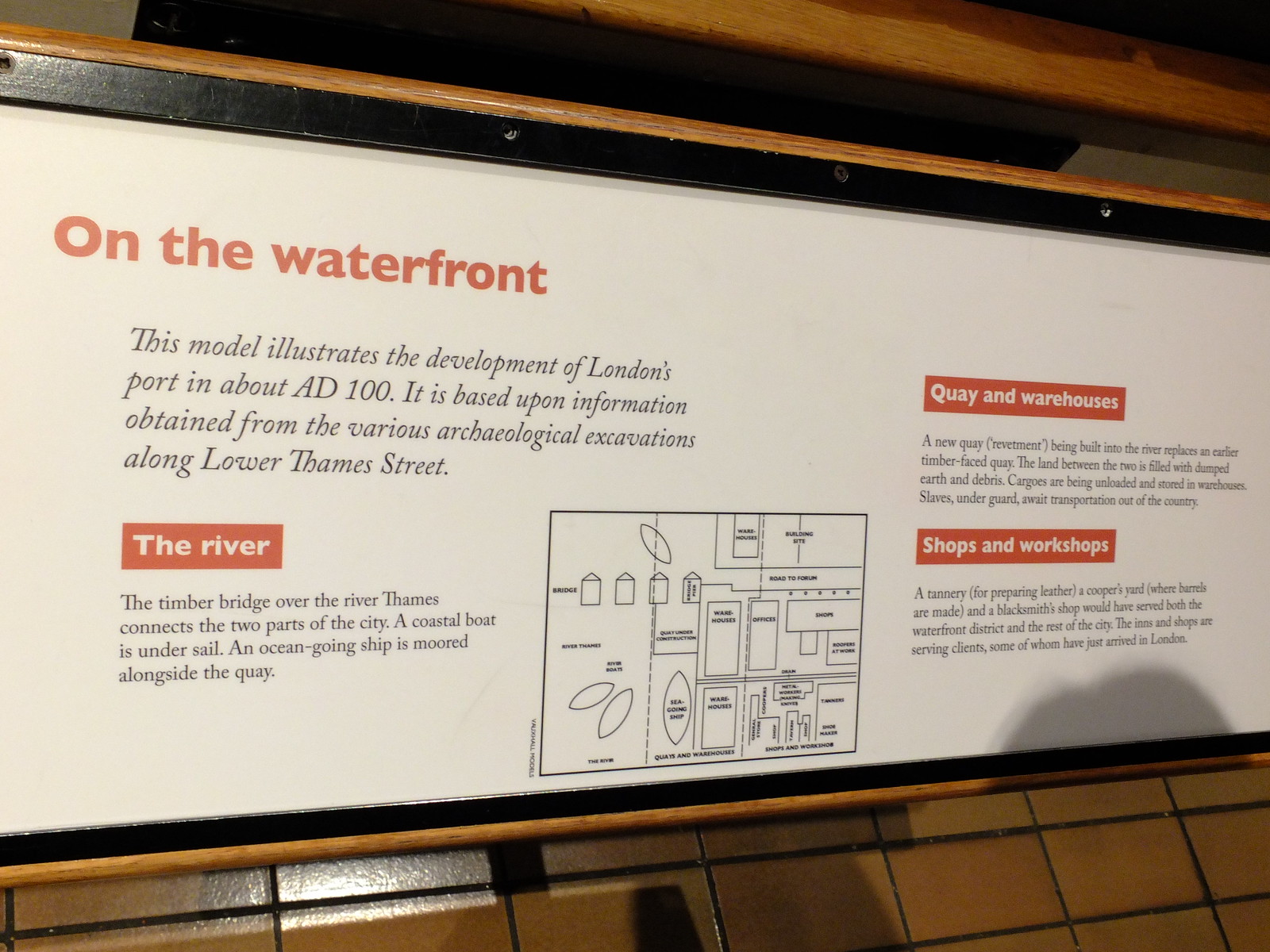The image depicts a museum exhibit featuring a horizontally oriented rectangular display, bordered in black with a wooden frame, mounted on a tiled wall in shades of tan, brown, and yellow. Dominating the center of the display is an illustrated sign with text in reddish-orange and black letters. The title "On the Waterfront" is prominently featured at the top in reddish-orange text. Below it, the black text details that "This model illustrates the development of London's port in about A.D. 100, based on information obtained from various archaeological excavations along Lower Thames Street." The illustration itself, set against a white background, depicts a historical scene with a timber bridge over the River Thames connecting two parts of the city, a coastal boat under sail, and an ocean-going ship moored alongside the quay. Additional text surrounds the illustration, providing further context and information. The setting appears to be indoors in a museum, hinting at an educational presentation of London's ancient port.